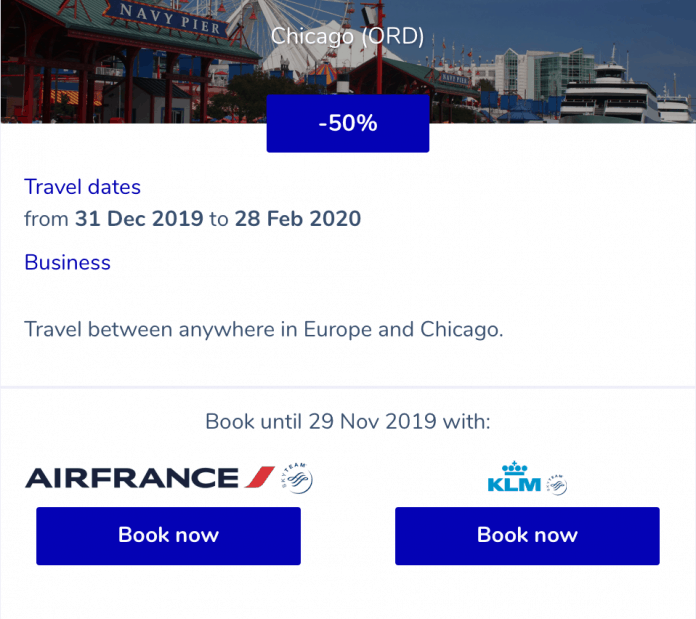This is a screen capture from a travel website, showcasing a promotional offer on airplane tickets. The main content highlights a discount for flights between Europe and Chicago O'Hare International Airport (ORD). Key details from the promotion include:

- A prominent blue button indicating a 50% discount.
- Travel dates available from December 31, 2019, to February 28, 2020.
- The promotion is labeled for business class travel.
- The offer applies for flights to and from various destinations in Europe and Chicago.
- Tickets must be booked by November 29, 2019.

The snapshot features the logos and booking options for two airline companies: Air France and KLM. The website, likely similar to platforms like Travelocity, provides options to secure these discounted fares, focusing on encouraging bookings between the specified dates and travel regions.